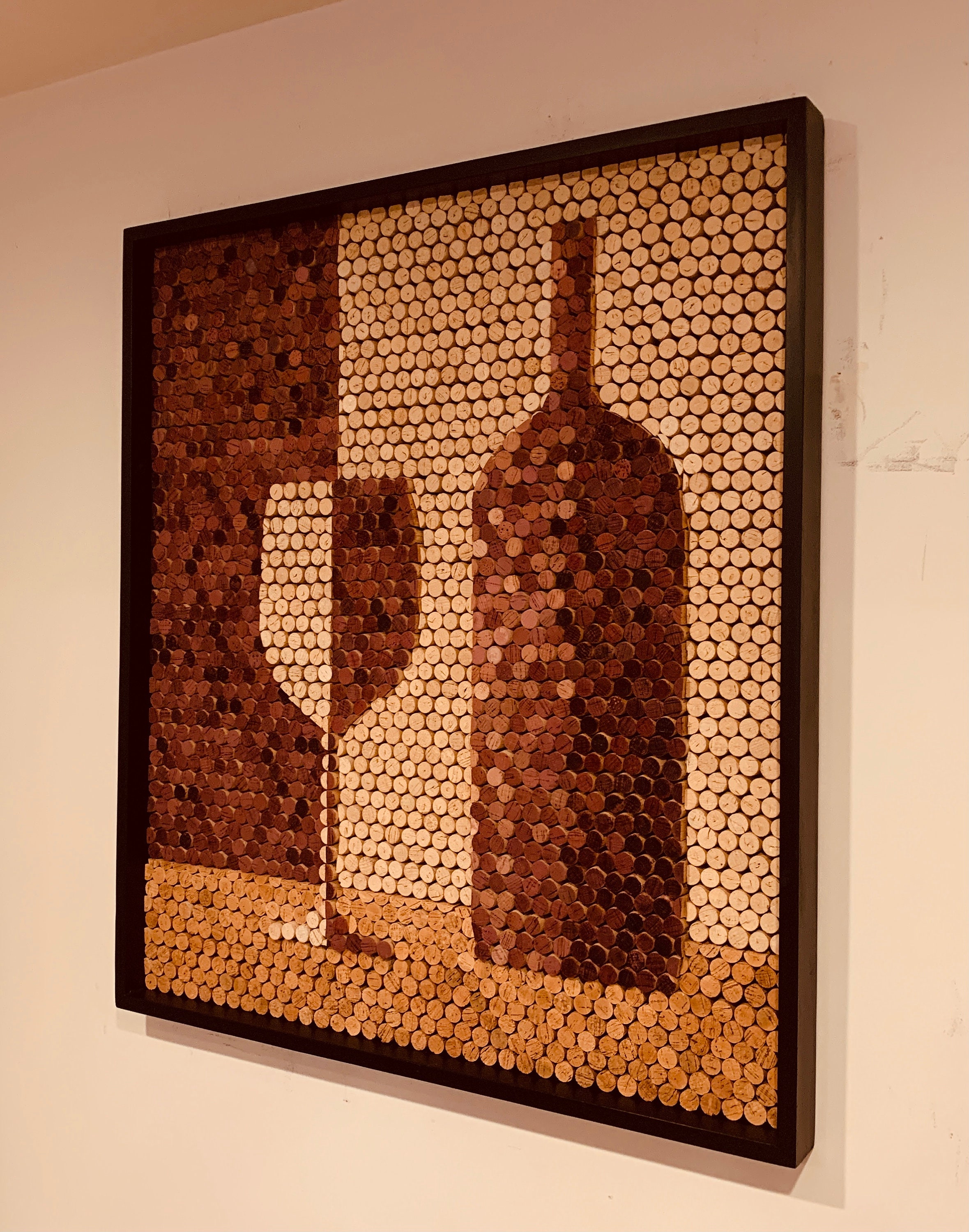The framed art piece mounted on a white wall, which has noticeable scuffs on the right side, features an intricate design made entirely of wine corks. Set in a sleek black frame, the artwork depicts a wine bottle and a wine glass, meticulously crafted to show depth and shading. The wine glass is composed of beige corks on the left and darker corks on the right, suggesting a play of light from the left side. Similarly, the wine bottle is rendered with darker brown corks on the right side, which also indicates shading and light source from the left. The background of the piece cleverly contrasts with the main subjects by using beige corks on the right and darker brown ones on the left. The corks are arranged both horizontally and vertically, and the varied colors range from beige to dark brown. The overall effect of the piece is a detailed and textured composition that vividly illustrates a wine bottle and glass, showcasing the artist's skill in using everyday materials to create compelling art.